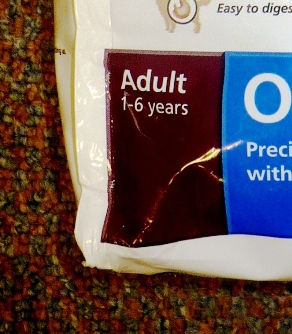The image captures a close-up of the bottom left corner of a white plastic package, possibly for dog food. The package is positioned on a colorful, spotty carpet featuring black, red, and yellow hues. Dominantly displayed on the package is a black rectangle with the white text "ADULT 1-6 YEARS." Beside it is a partially visible blue rectangle, also containing white text, beginning with "0 PRE" and partially obscured. Above the text sections, there is an incomplete silhouette of an animal, presumably a dog, with the accompanying text "EASY TO DIGEST." The photograph provides a highly zoomed-in view, prominently showcasing these textual details.